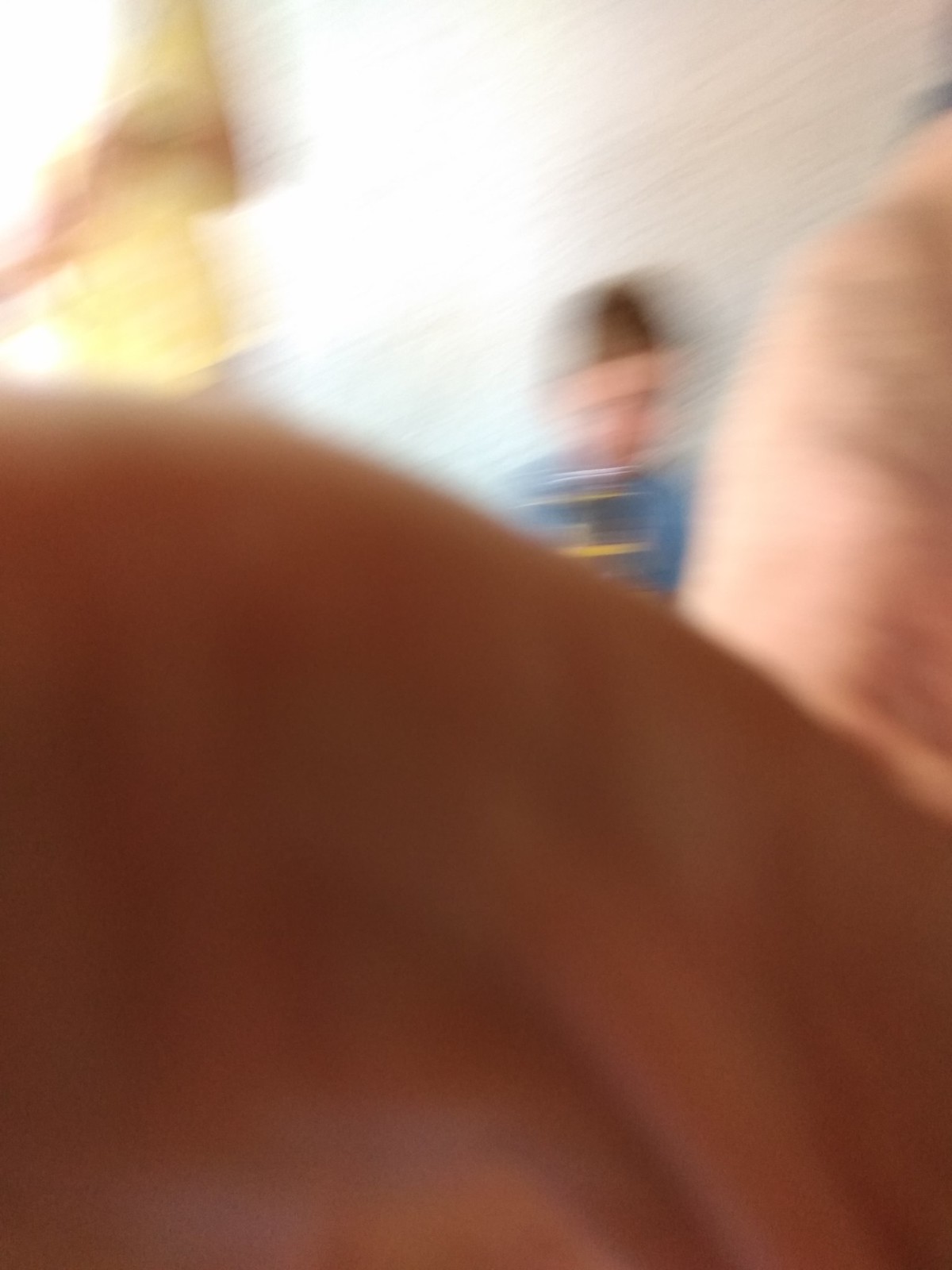In this photograph, which is notably out of focus, the majority of the frame is dominated by a large hand, possibly obscuring the camera lens by mistake. The hand, likely belonging to the person taking the picture, occupies approximately two-thirds of the image and shows visible wrinkles, suggesting age or close-up detail. To the right side, a thumb can be discerned, adding to the impression of accidental coverage. Beyond the hand, the hazy outline of a child emerges, characterized by short dark brown hair and a light blue shirt with streaks of yellow. Although blurry, the backdrop seems to feature a white painted wall, indicative of a home setting. The overall blurriness suggests the photo was taken in motion or perhaps just before or after the camera was dropped.